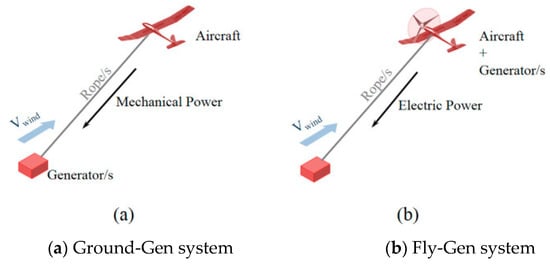The image features two schematic illustrations side by side labeled "A" and "B," depicting different aircraft power generation systems. 

On the left, "A" is labeled "Ground Gen System." It shows a red aircraft situated mid-air connected to a red 3D box labeled "Generator" on the ground by a gray cord marked "Ropes." An arrow labeled "Mechanical Power" points downward from the aircraft to the generator. Additionally, a blue arrow labeled "V1" points upwards.

On the right, "B" is labeled "Fly Gen System." This illustration shows an aircraft labeled "Aircraft + Generator" with a propeller indicating its self-propulsion. Below it is a box with an arrow pointing downwards labeled "Electrical Power." Unlike "A," this system integrates the generator with the aircraft itself for power generation.

Both illustrations use similar visual elements and color schemes to differentiate between the two systems of mechanical versus electrical power generation in aircraft.